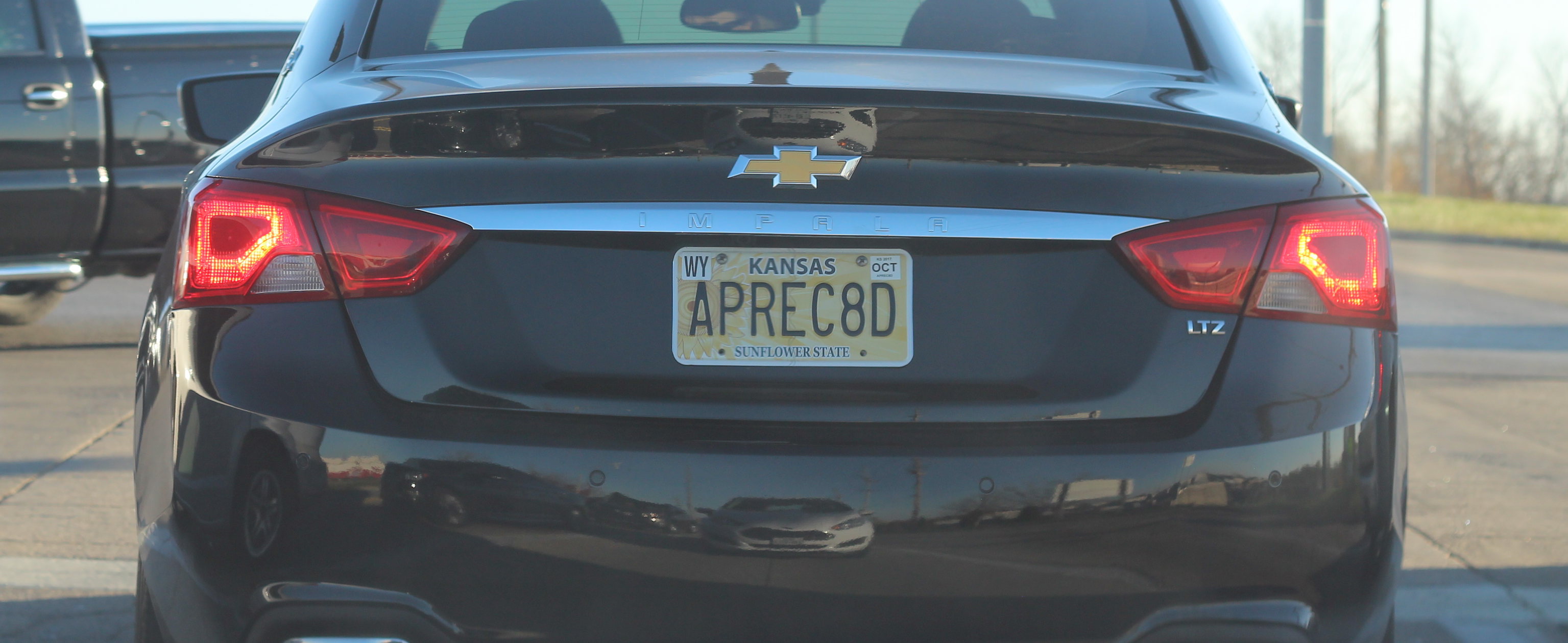This image, a narrow horizontal close-up twice as wide as it is tall, captures the rear of a dark blue Chevrolet Impala LTZ on a late afternoon, with the taillights illuminated as if someone is pressing the brakes. The vehicle, which features tinted windows, spans the width of the frame from the lower part of the rear window to just below the bumper. Prominently displayed in the center of the trunk is the Chevrolet cross symbol, positioned above a yellow Kansas license plate with the personalized text "A-P-R-E-C-8-D," translating to "appreciated." The plate also carries a small W-Y sticker in the left corner and an O-C-T sticker in the right, indicating the registration renewal month. Additionally, the model designation "LTZ" is visible in small letters on the right side of the trunk, and the image includes a faint reflection of a silver car in the vehicle's glossy surface. The scene suggests it is a sunny day with the sun beginning to set.